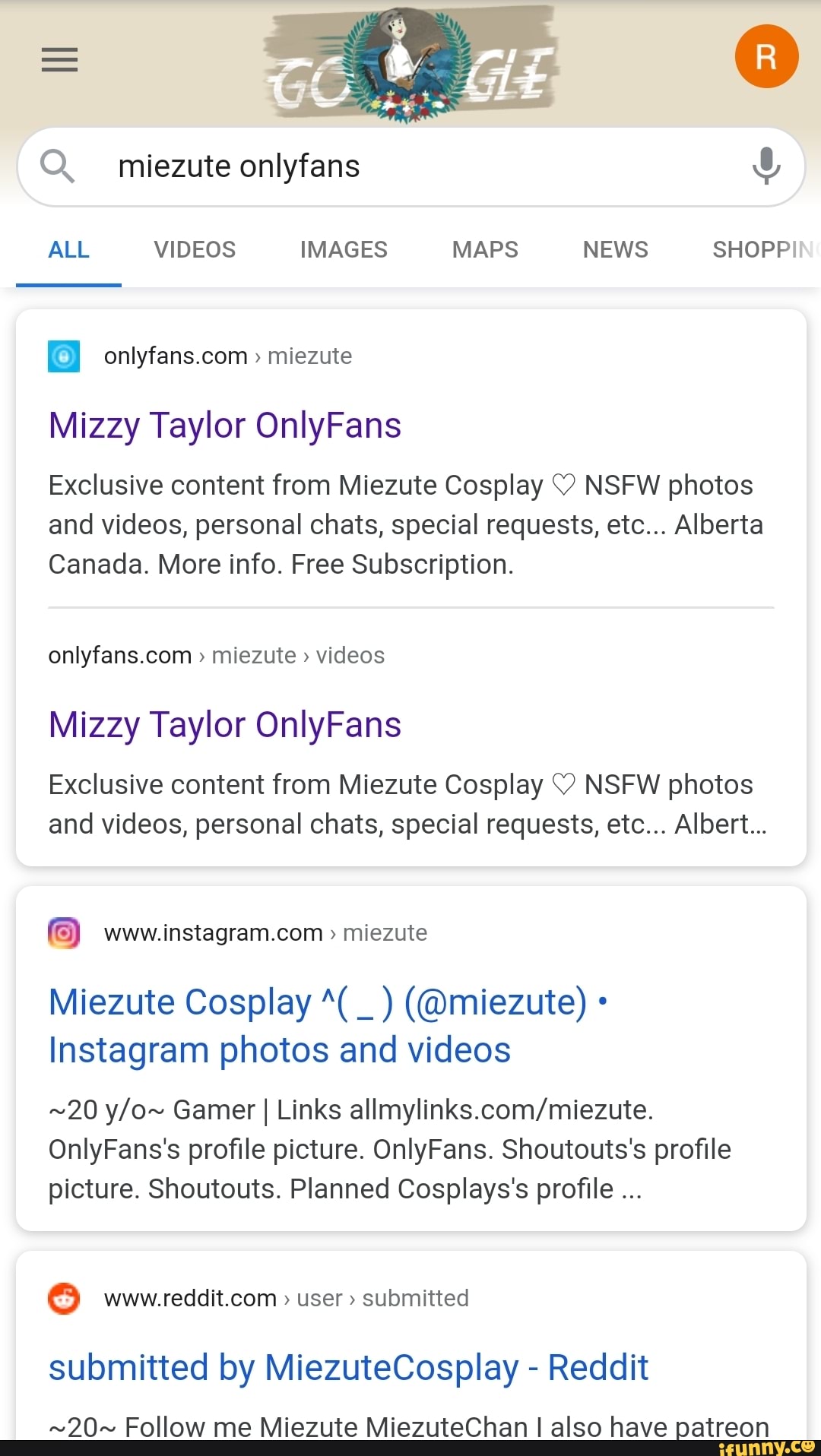The image is a screenshot from someone's phone, displaying a vertical rectangle. At the top, the Google search interface is visible, with Google's second 'G' transformed into a stylized person surrounded by flowers. In the upper right corner, there is an orange circle featuring a white 'R'. Below, in the search bar indicated by an oval containing a magnifying glass icon, the text "MIEZUTE" is entered, accompanied by the additional text "MeZoot Only Fans."

At the top left of the search results, the "All" category is selected and underlined in blue. The search results listed below include the following:

1. First result: "OnlyFans.com" with the subtitle "Mizzy Taylor Only Fans."
2. Second result: "OnlyFans.com" repeating "Mizzy Taylor Only Fans."
3. Third result: An Instagram link with the logo, stating "Instagram.com, MeZoot Cosplay" along with a description referring to Instagram photos and videos.
4. Fourth result: A Reddit link showing the text "submitted by MeZoot Cosplay Reddit."

Overall, the search query "MeZoot Only Fans" was entered into Google, and these are the corresponding search results displayed on the screen.